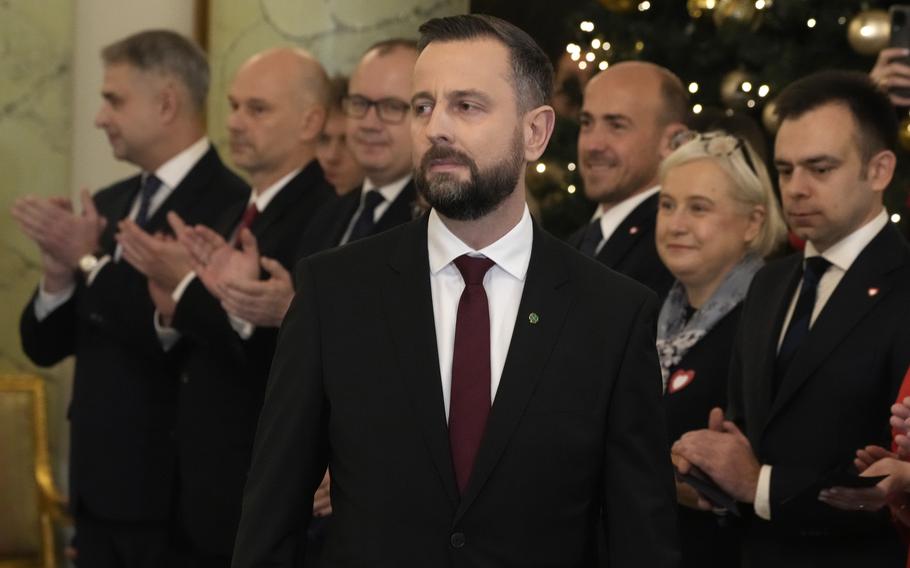In the image, a well-dressed man stands prominently in the front center with a neutral to negative expression, his gaze directed to the side. He has short dark hair, a beard, and a mustache. He is wearing a black suit jacket adorned with a pin, a white shirt, and a maroon tie. Surrounding him are six other individuals, all dressed formally in black suits with white shirts. To his left, a man in a black suit with a white shirt and a wristwatch claps his hands. Next to him is a mostly bald man with a mustache, also in a black suit with a red tie, clapping. Another man with very short hair, wearing glasses, and a black suit claps to the right of the bald man.

To the right of the central man is another individual with very short hair, mustache, and beard, also in a suit with a dark tie and a pin. Beside him stands a blonde woman with short hair, smiling faintly, wearing glasses perched on her head, a dark suit, a lighter blue-gray scarf, and a red pin. On her right, a man in a dark suit with a white shirt and a pin claps his hands. 

The group appears to be applauding, though all are looking in different directions, suggesting the applause is not directed at the central man. The image is set indoors, possibly at a business event, as indicated by their formal attire and the presence of ornaments or lights in the background. The expressions among the group vary, with some individuals smiling while others maintain neutral expressions.